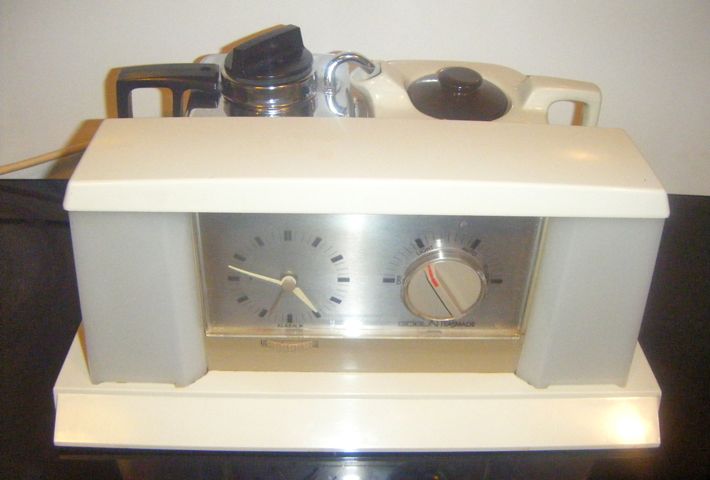The image is a color photograph of what appears to be a modern, retro-styled appliance, possibly an old-style automatic coffee maker or a clock with a timer. The main device is rectangular and predominantly white, likely made of plastic, with smooth surfaces and two thick pillars on either side. The front features a stainless steel panel, with a gold-bordered, numberless clock displaying black rectangles to represent hours and gold hands, including a second hand. To the right of the clock is a plastic dial with four black rectangular sections indicating different settings, and a red marker for selection.

The device sits on a tabletop, which is either black or very dark brown. Behind the main appliance are two additional objects: one on the left with a shiny silver top, black handle, and black lid, likely a pot; the other resembling the main appliance's material with a circular brown lid or handle. The background includes a partial view of a white wall on the top two-thirds of the image and portions of the tabletop on the lower section. An electrical cord is seen on the left side, hinting at the appliance's connectivity.